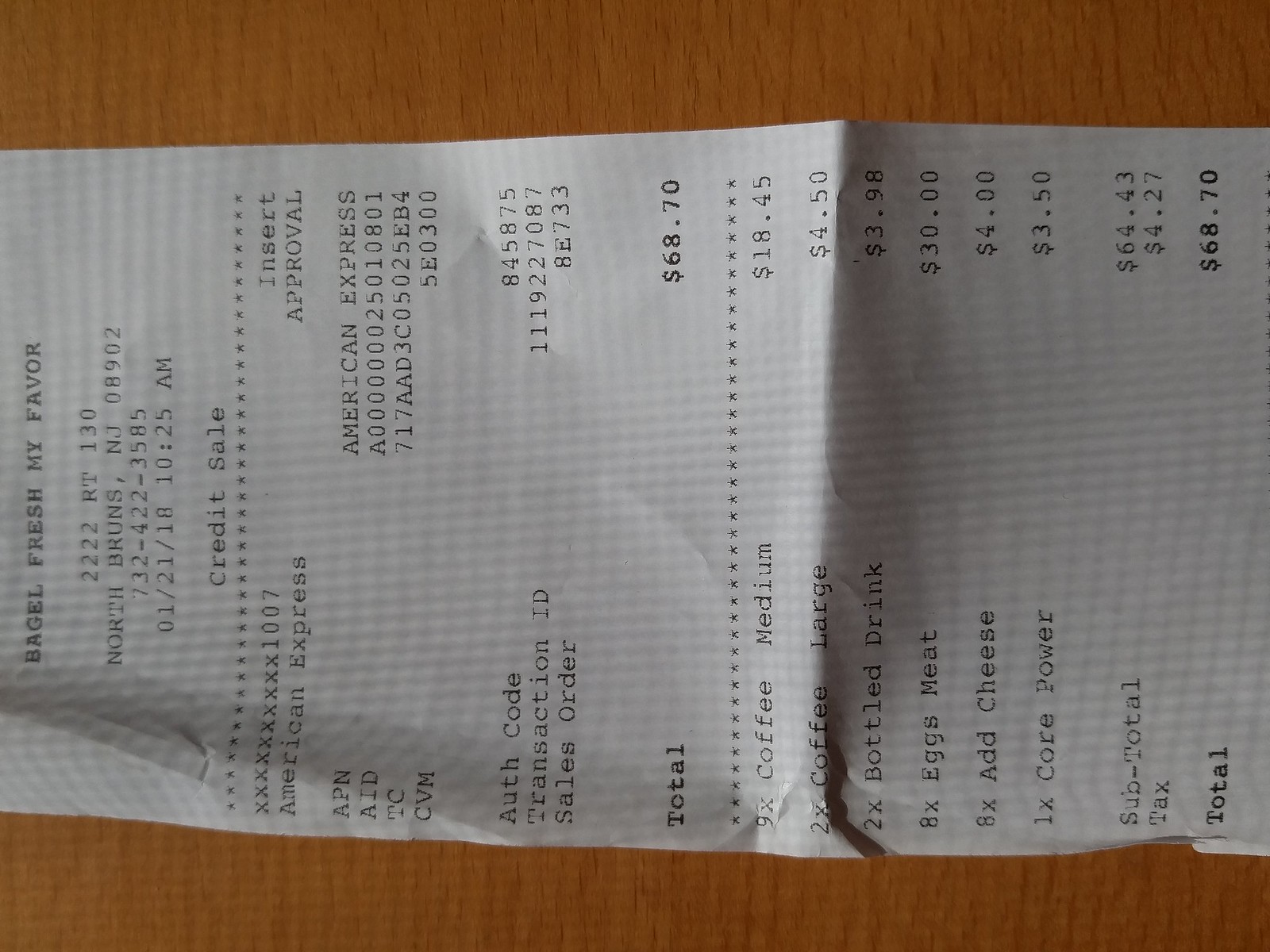This is a detailed photograph of a receipt from Bagel Fresh, my favorite bagel shop, located in North Brunswick, New Jersey. The image captures the intricate details and itemization on the receipt, reflecting the purchases made.